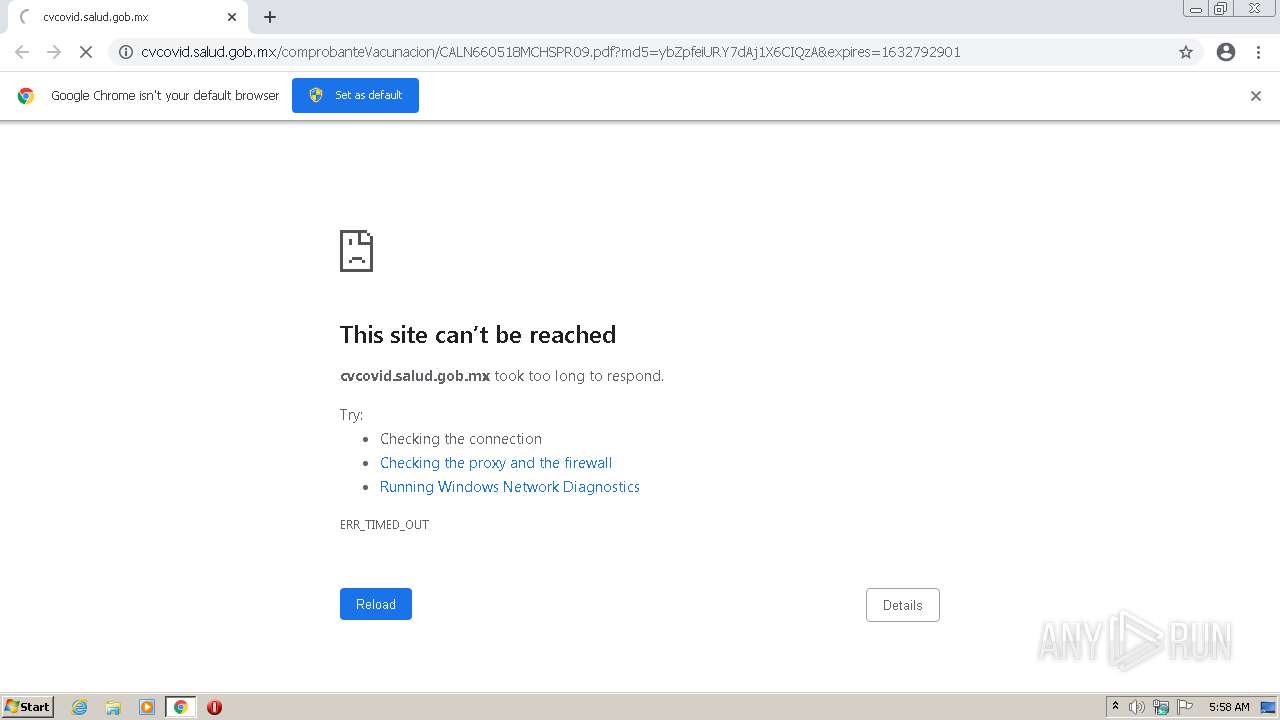A screenshot captures the desktop of a computer running Windows 7 in classic mode, identified by the distinct style of the taskbar. The focal point of the image is a Google Chrome browser window open to the website "cvcovid.salud.gob.mx". A prominent notification at the top informs that Google Chrome is not set as the default browser, providing an option to change that.

The browser window displays an error page with the message "This site can't be reached." The error icon accompanies the text stating, "cvcovid.salud.gob.mx took too long to respond. Try checking the connection, checking the proxy and the firewall, running Windows Network Diagnostics. ERR_TIMED_OUT." At the bottom of this message, "Reload" and "Details" buttons are visible for further action.

The taskbar, timestamped at 5:58 AM, includes icons for sound, notifications, and various applications: Chrome browser, Opera browser, Windows Media Player, File Explorer, and Internet Explorer. The classic Start button is also present. A watermark in the bottom right corner reads "AnyRun," indicating the use of this security analysis tool.